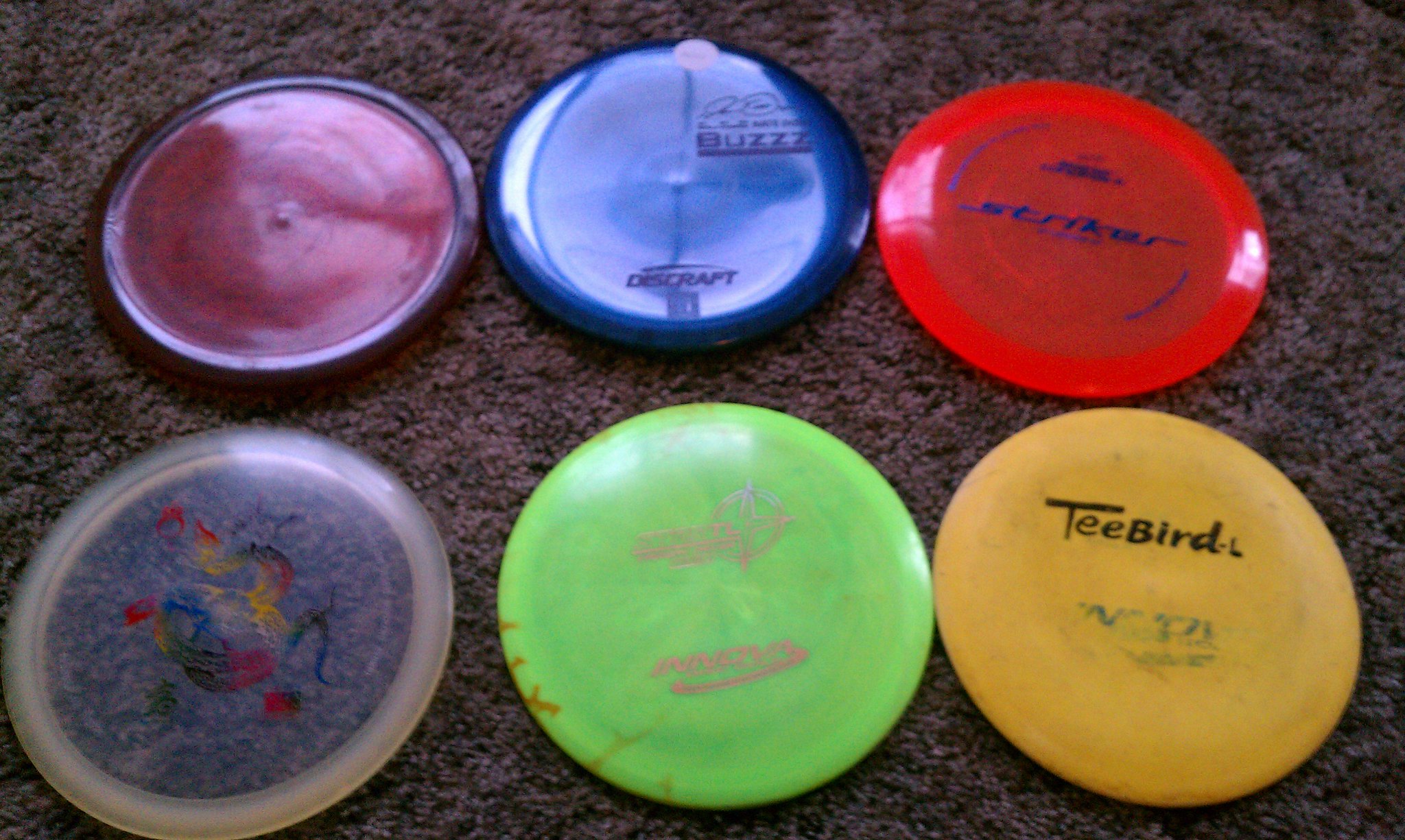The image features six frisbees arranged on a dark gray carpet. The frisbees vary in color and condition. The first frisbee, on the top left, is yellow with the word "T-Birds" printed on it; it appears quite old, dirty, and worn. Next to it is a lime green frisbee with indistinct words, as the writing is flushed out by the color. The center frisbee in the arrangement is clear, allowing the carpet's pattern to show through. Adjacent to this is a pinkish-purple frisbee with a solid color and a purple rim. The next frisbee is shiny blue and looks new, bearing the words "Buzz" and "Disc Craft." Lastly, on the top right, there is a red, see-through frisbee with the word "Striker" written in blue.